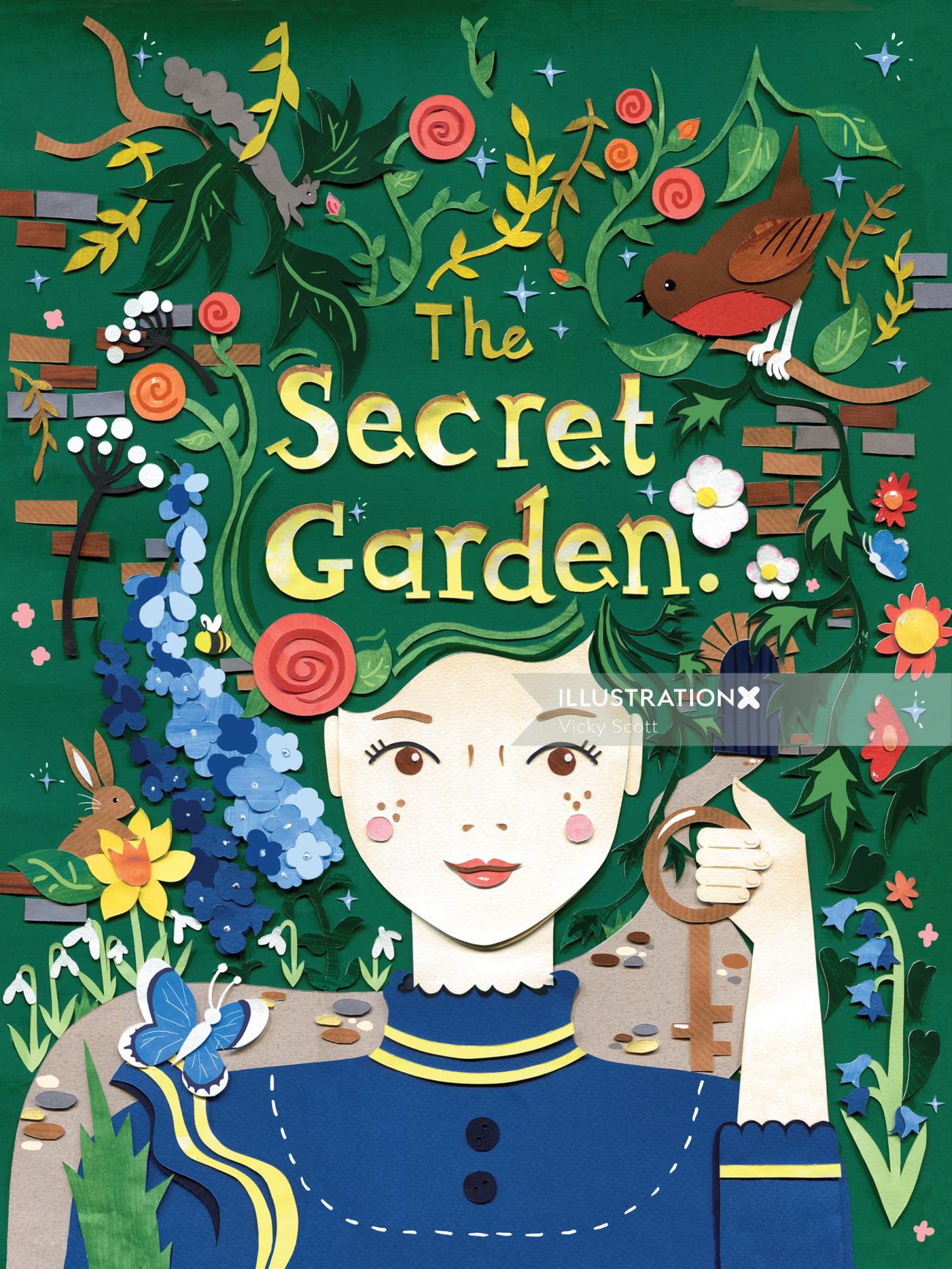The image is a detailed, color illustration resembling a book cover for "The Secret Garden," executed in a paper-cut style. Against a vibrant green background teeming with an array of plants, animals, and intricate designs, "The Secret Garden" is prominently displayed in gold and yellow letters in the upper central portion. The top half of the artwork is adorned with various colored plants, including green, pink, and gold flowers, as well as light and dark brown bricks accentuated with light purple hues. A singular robin, characterized by its brown feathers and yellow-red stomach, perches on a tree branch amidst this botanical chaos.

Below the title, a young woman stands facing the viewer. She features pink freckles across her white face and is dressed in a high-necked blue blouse accented with yellow details and two black buttons. Her green hair merges seamlessly into the surrounding floral imagery, creating an enchanting integration of the character with the garden's essence. In her left hand, she clutches a large brass key, suggesting a critical element of the story. A blue butterfly delicately rests on her right shoulder, complementing the array of blue flowers and a singular yellow blossom nearby. There is a subtle watermark on the illustration that reads "Illustration X, Vicki Scott." All these elements together create a captivating visual summary of the enchanting world within "The Secret Garden."